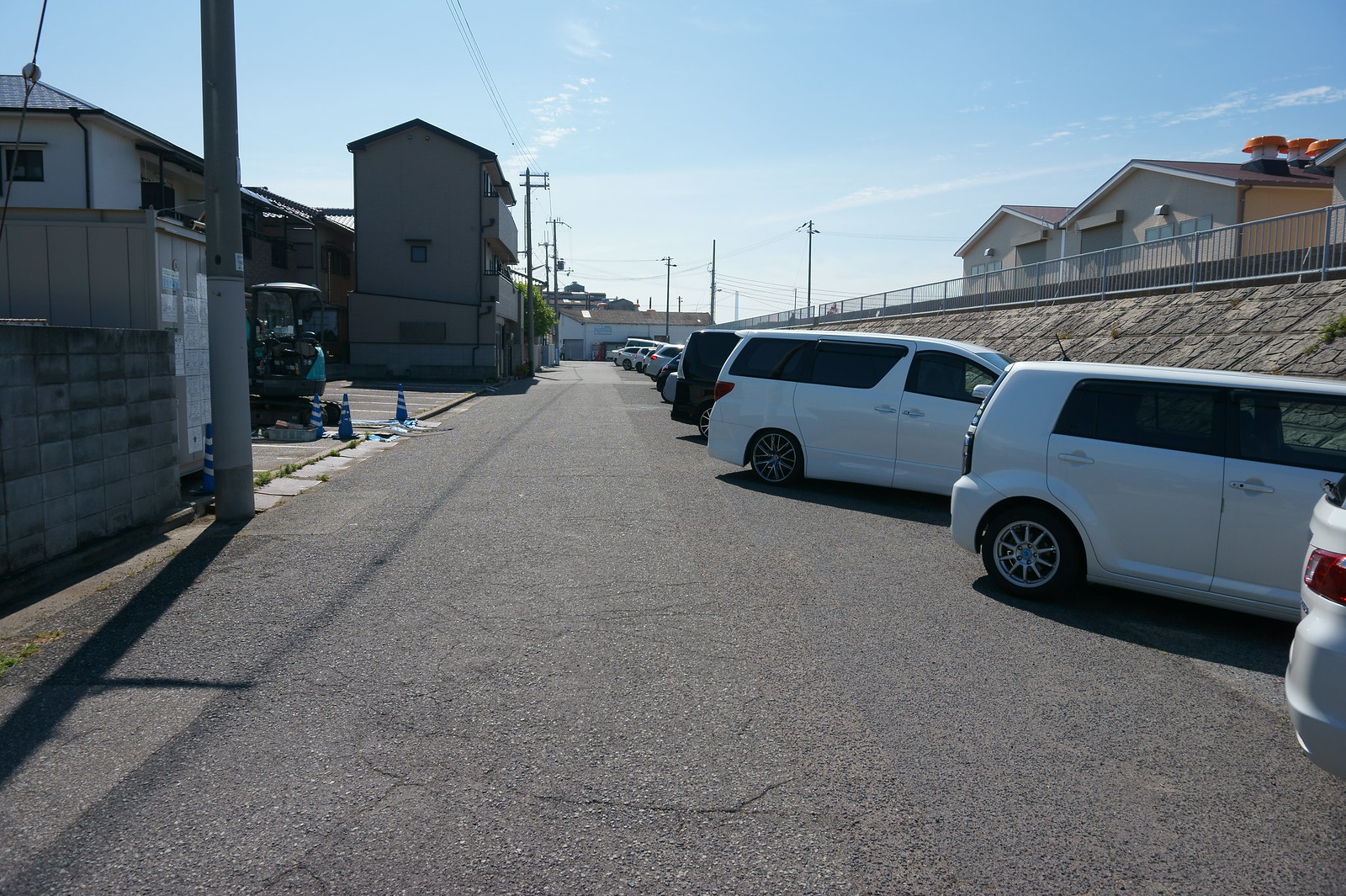This detailed photograph captures a narrow, paved alleyway serving as a parking lot in what appears to be a residential neighborhood. The alleyway, widest towards the back and narrowing as it extends to the middle horizon, is lined with diagonally parked cars, including a white SUV or van, another white van, and a black van closest to the camera. The plain gray concrete of the alleyway shows fine cracks near the bottom of the frame, and there are no visible lines dividing up the parking spots. On the left side of the image, three-story apartment buildings stand prominently, with one positioned closer to the camera and two others arranged perpendicularly in the far background.

A tall utility pole is situated in the top left corner of the photo, adding to the urban feel of the setting. Between the closer apartment building and the alleyway, a piece of teal-colored construction equipment is visible. To the right of the alleyway, a steep embankment rises, topped by a gray metal barrier. Beyond this barrier, two beige houses can be seen, flanking a paved road behind the fence. Additional homes and buildings extend into the background, giving a sense of depth and community.